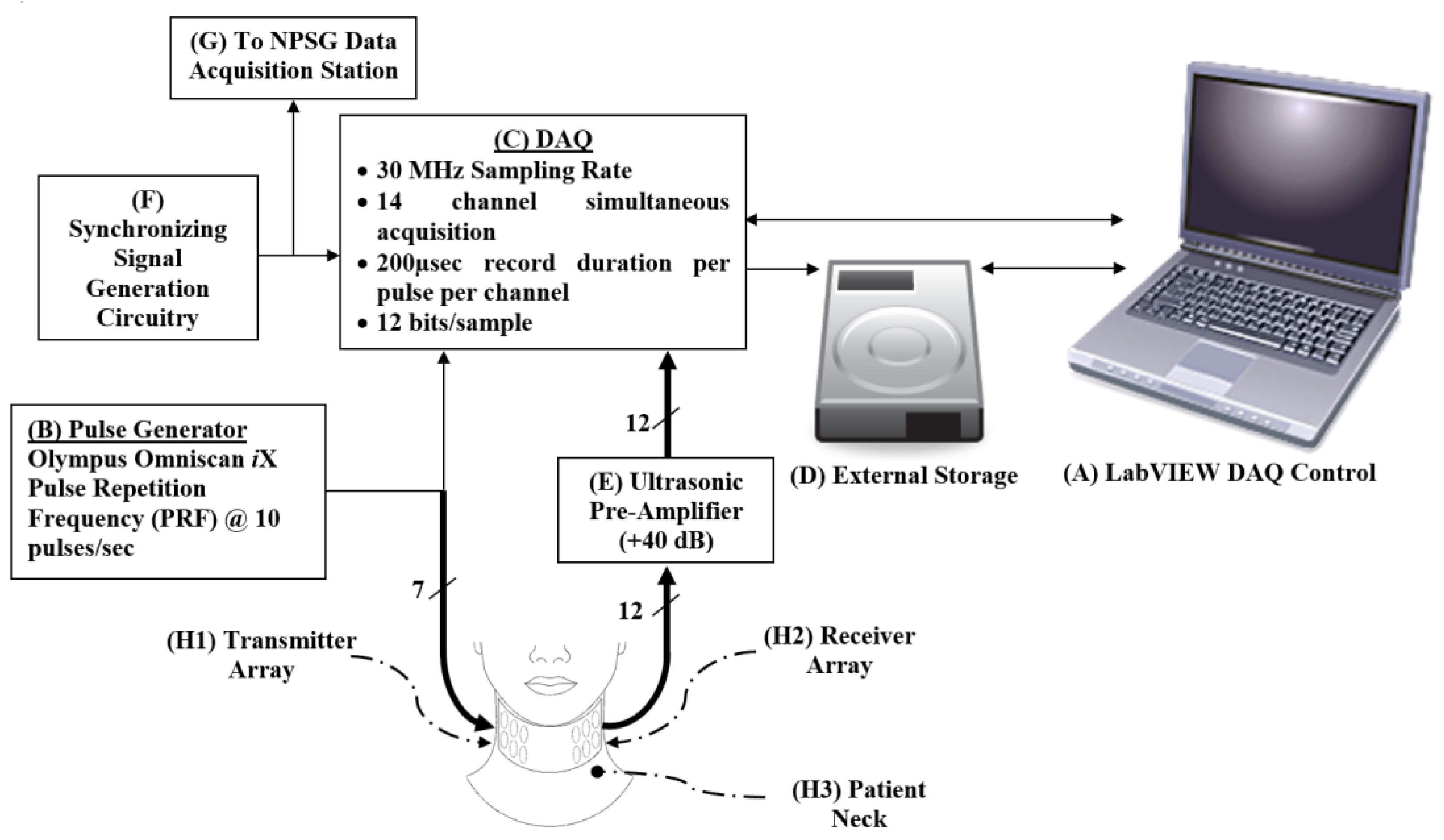The image is a detailed diagram illustrating a pulse monitoring and correction system integrated with a laptop computer. At the center top of the diagram, the laptop is prominently labeled "A - LabVIEW DAQ Control," indicating its role in the data acquisition and control process. The laptop interfaces with various components through "B - Pulse Generator Olympus Omniscan IX" which operates at a pulse retention frequency of 10 pulses per second. 

Inputs and outputs are shown with labels ranging from B through H3, involving complex interactions. Located at the bottom of the image is a schematic of a patient's head and neck, showing only the lower parts including the nose, mouth, neck, and lower ears. This section highlights the "H1 - Transmitter Array," "H2 - Receiver Array," and "H3 - Patient Neck." Data from these arrays are processed through "E - Ultrasonic Preamplifier (+40 dB)" and transmitted back to the laptop. 

The laptop is additionally connected to "C - DAQ," which is specified as having a 30 megahertz sampling rate and a 14-channel simulation acquisition capability, along with "D - External Storage" to save the collected data. The system also incorporates "F - Synchronizing Signal Generation Circuitry" and routes data through "G - NPSG Data Acquisition Station," demonstrating a comprehensive setup for monitoring, acquiring, and processing pulse-related data in real-time.